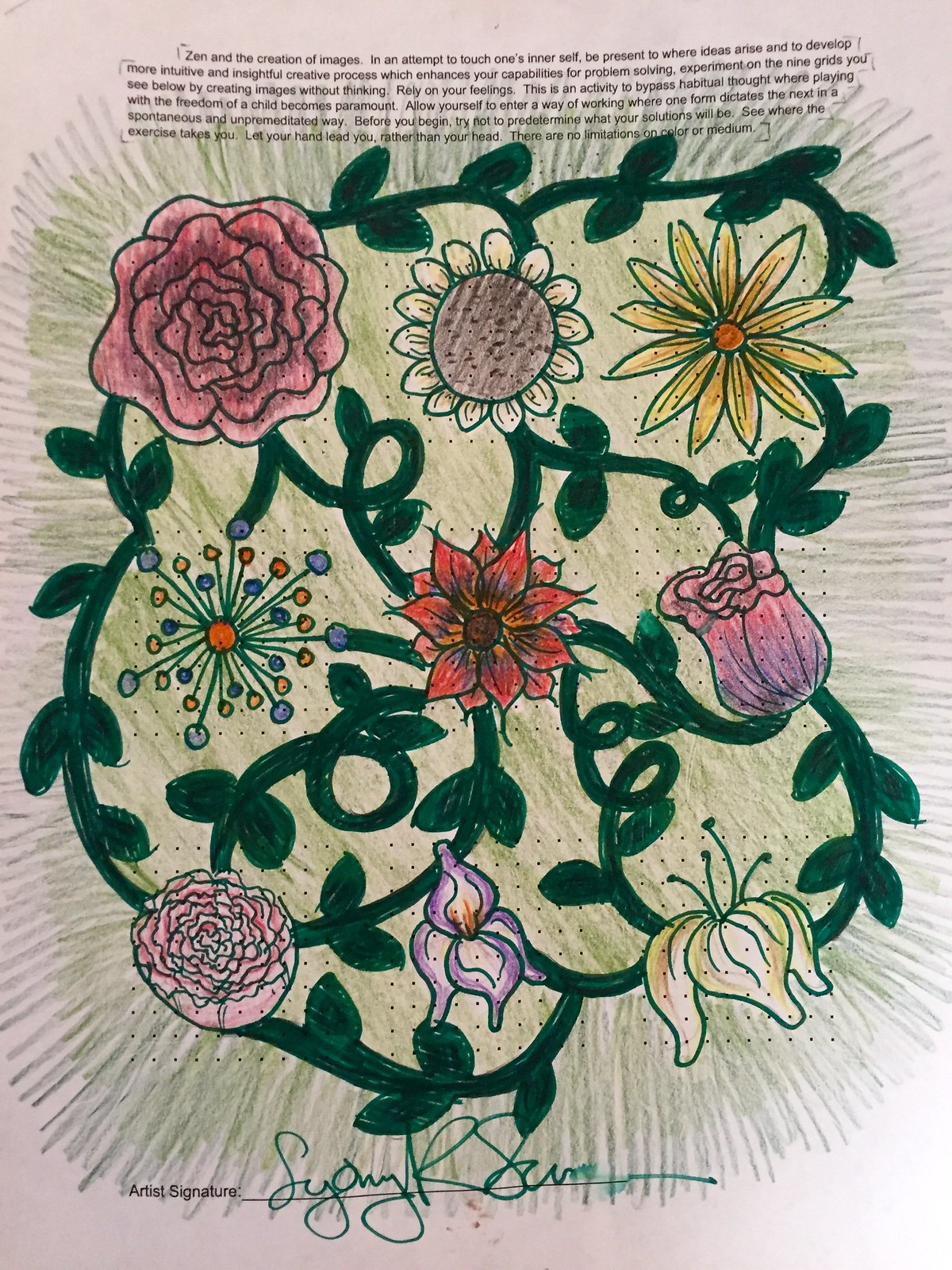The image is a detailed floral drawing, signed by the artist Sydney R. The text at the top describes a Zen-inspired creative process urging one to touch their inner self and develop intuitive and insightful problem-solving skills. It instructs the viewer to experiment on nine grids below by creating images without thinking, relying on feelings to bypass habitual thought and embrace the freedom of a child. The drawing itself features interconnected colorful flowers, including pink carnations, yellow sunflowers, blue daisies, and orange tulips, all entwined by a thick green vine adorned with leaves. The exercise encourages spontaneous and unpremeditated creation, allowing forms to dictate the next in a flow led by the hand rather than the head.